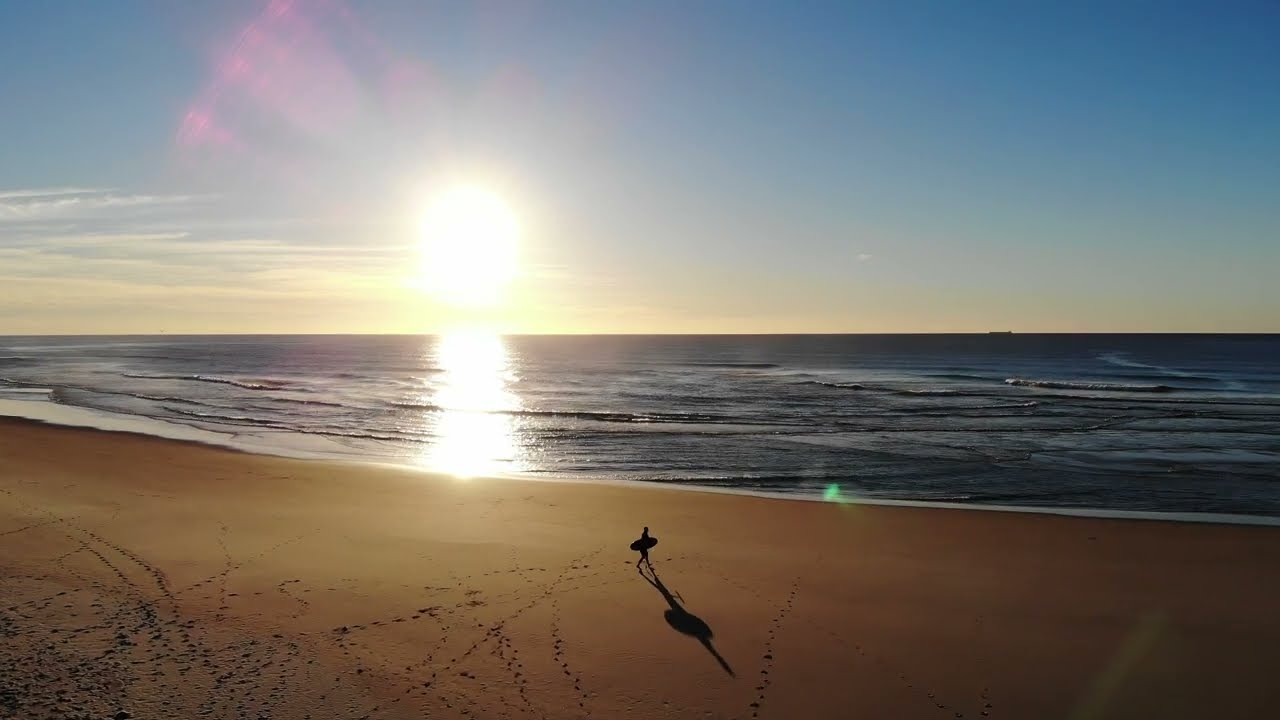At a tranquil beach scene, likely at the break of dawn or twilight, the landscape is primarily dominated by serene browns of the sand in the foreground and contrasted by the calming blues of the ocean and sky. The sky, mostly clear with a few horizontal clouds, boasts a low-hanging Sun, casting a radiant yellow-glow and a subtle pinkish hue across the scene. The Sun’s reflection creates a golden band shimmering on the water's surface. Although the beach is empty, numerous footprints dot the sand, hinting at earlier activity. Central to the image, yet distant, is a solitary figure heading towards the calm, almost wave-less ocean, carrying a surfboard under their arm. Their shadow stretches along the shoreline, amidst patches of foamy white water contrasting the distant darker, choppier sea.